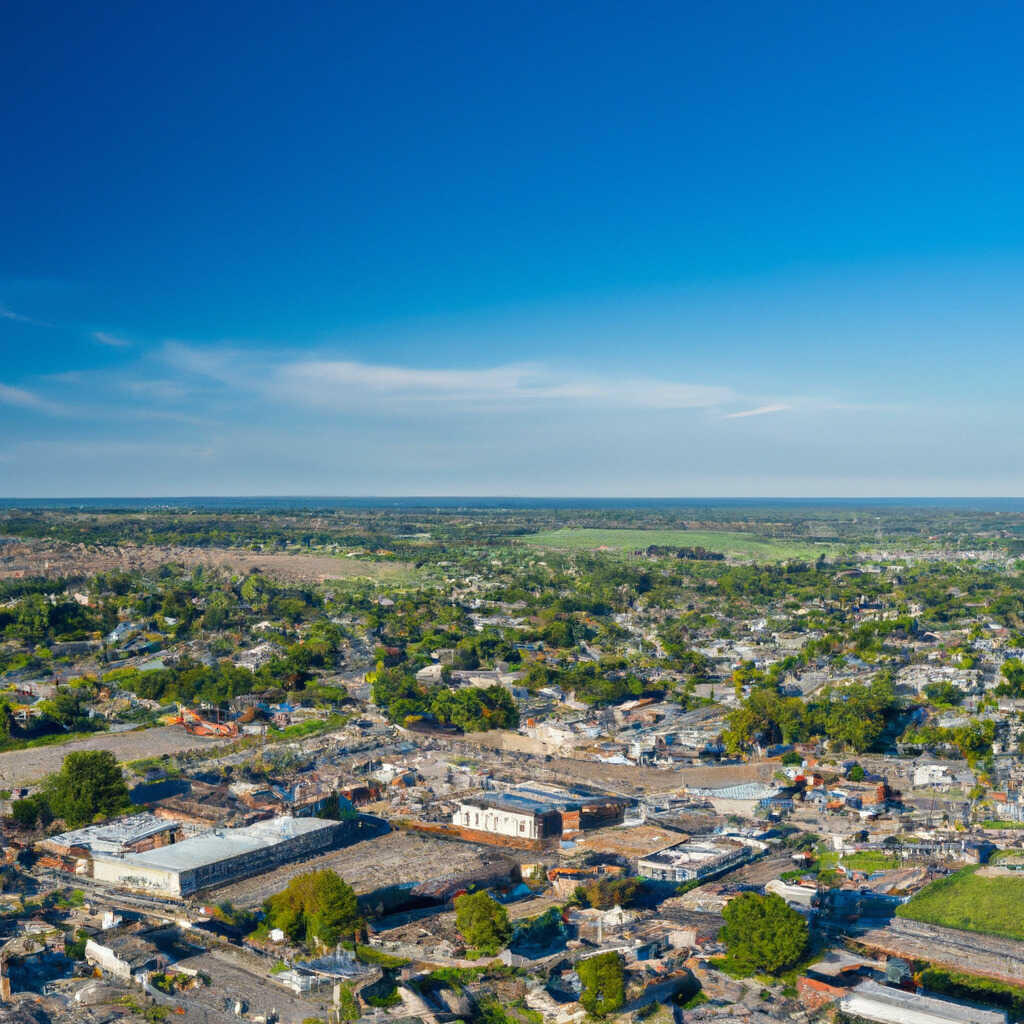This image, likely an altered and oversaturated photograph originally scanned and enhanced in Photoshop, provides a sprawling aerial view of a metropolis with a distinct horizontal division. The top third of the image showcases a deep blue sky, transitioning to lighter hues near the horizon, punctuated by long, wispy white clouds. Below this, a strip of dark blue water—possibly an ocean—forms a clear demarcation before giving way to the cityscape. The city's buildings predominantly appear gray or white, varying in architectural forms from flat, rectangular rooftops on the left to two-story masonry structures. Throughout the city, vibrant green vegetation, including full green trees and expansive grassy fields, is interspersed among the buildings, creating pockets of natural beauty within the urban landscape. The overall image may not be entirely in focus, further emphasizing its altered photographic quality.